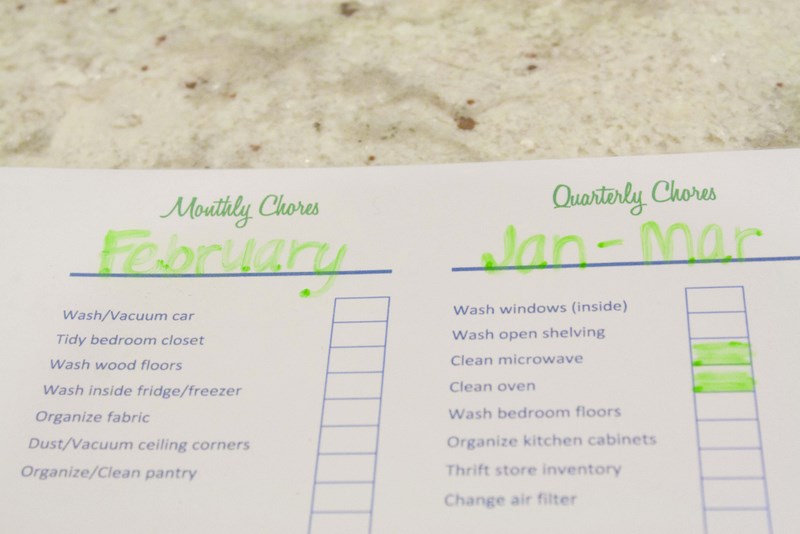This photograph captures a detailed chore checklist placed on a countertop with a gray marble appearance and brown specks. The list is divided into two sections: "Monthly Chores" and "Quarterly Chores." The "Monthly Chores" section, labeled in green under "February," includes tasks such as washing and vacuuming the car, tidying the bedroom closet, washing wood floors, washing the inside of the fridge and freezer, organizing fabric, dusting and vacuuming ceiling corners, and organizing and cleaning the pantry. To the right, the "Quarterly Chores" section for January to March, also written in blue, lists tasks like washing windows inside, washing open shelving, cleaning the microwave and oven, washing bedroom floors, organizing kitchen cabinets, taking thrift store inventory, and changing air filters. Both sections feature a grid style with checkboxes to track progress; currently, only the tasks of cleaning the microwave and oven are marked with green checkmarks.